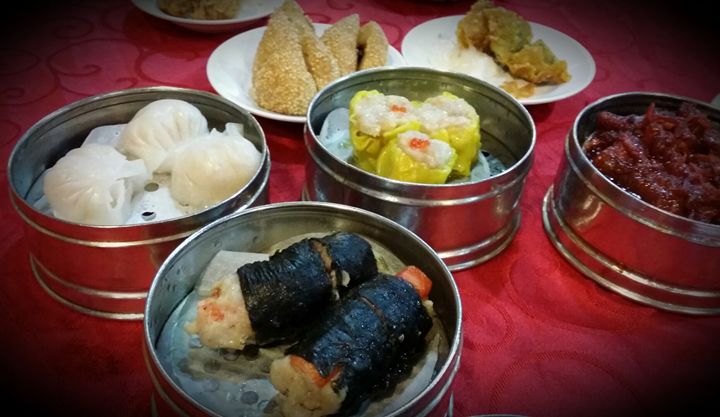The image features an assortment of silver, shiny, metal containers, each devoid of lids, revealing various intricate food items inside. All of this rests atop a rich, velvety red tablecloth adorned with delicate filigree patterns. The photo is taken from a perspective that looks down and across the tabletop. Among the containers, one holds seaweed-wrapped pieces akin to crab or lobster sushi rolls. Another contains semi-transparent white dough intricately folded around a round filling, resembling dumplings. A third container houses wrinkled yellow bell peppers, stuffed with a mixture of rice and a red substance. The fourth container is filled with cranberry jelly, its deep red hue standing out. Behind these containers are three white plates, each bearing fried food items, likely including rice. The leftmost plate seems to feature breaded items, while the rightmost presents with brown-tinted food, completing this visually diverse and intricate culinary display.